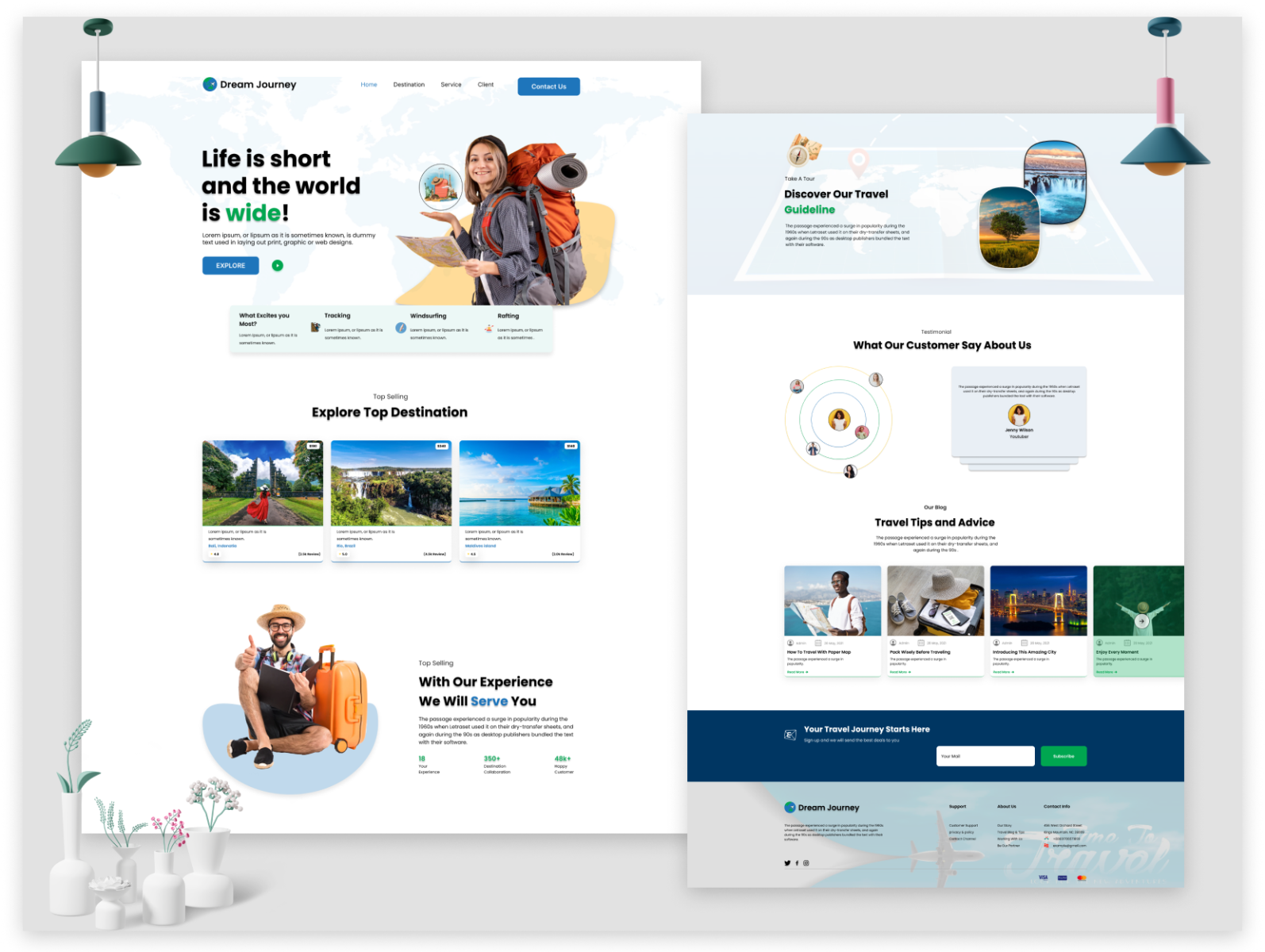A screenshot captures a proposed webpage layout, encapsulating the adventurous theme "Life is short, the world is wide." The upper section showcases a series of vibrant images depicting various travel destinations against a sleek gray background. Below these images lies a layout, hinting at the website's design, which includes a blue bar at the bottom of the screen. This bar features a sign-up field for a newsletter, encouraging user engagement. Additionally, global navigation options are elegantly positioned at the very bottom of the page, ensuring easy site-wide accessibility.